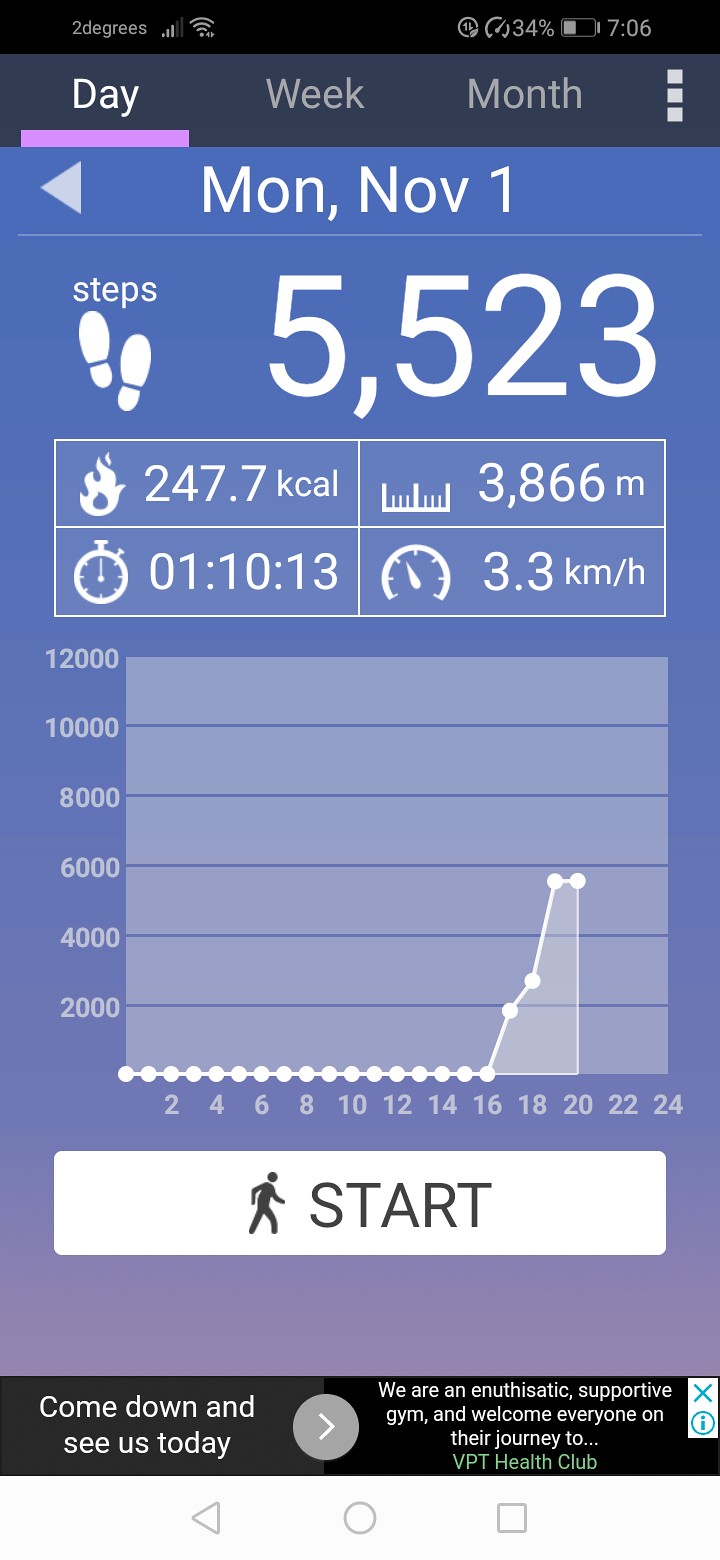This image is a vertical rectangular screenshot from a step-tracking app displayed on a cell phone. The screen is predominantly blue, gently transitioning to purple towards the bottom, with white text throughout. At the very top, there's a black status bar containing cell phone navigation indicators like time and date. Just below this bar, the app features three toggle options labeled "day," "week," and "month," with "day" currently selected. Underneath this, the current date, "Monday, November 1st," is prominently displayed in white text.

The main section of the screen showcases the step count, "5,523 steps," accompanied by a graphic of two shoe prints. Additional details include calories burned (247.7 kcals), distance walked (3,866 meters), duration (1 hour and 10 minutes), and average speed (3.3 km/h), all presented in white against the blue background.

Below these statistics is an XY graph charting the steps taken over time, with markers indicating intervals of 2,000 steps, peaking at 12,000 steps. The horizontal axis likely represents the days of the week. At the very bottom of the screen, a black button labeled "Start" is positioned next to an icon of a human figure, enabling the user to begin a new tracking session.